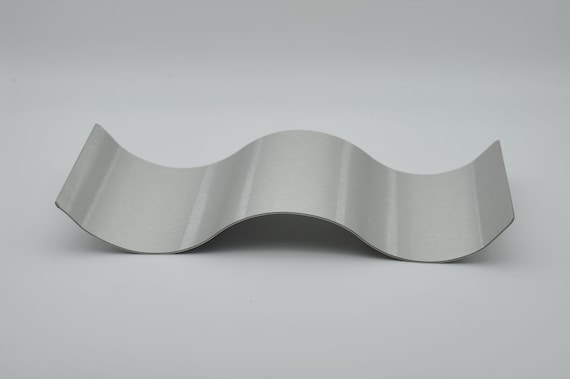The image features a piece of metal, likely stainless steel, with a brushed finish, intricately designed into an S-curve or wave shape. The metal displays a gradient of gray shades running horizontally across its surface, with four distinct bands being slightly darker. Measuring approximately 15 inches long and 8 inches wide, this rigid piece seems prone to snapping if bent further. It rests on a white, matte, shiny table surface, casting darker shadows beneath its curves. The photograph is captured from above at a slight angle, emphasizing the undulating wave form and the subtle variations in its brushed gray finish.